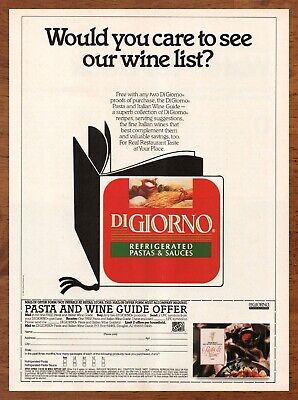This image is a vintage magazine advertisement featuring DiGiorno refrigerated pastas and sauces. Resting on what appears to be a wooden table, the ad is framed by a thin brown border. At the top, in black text on a white background, it asks, "Would you care to see our wine list?" Below this question is a block of small, unreadable text. The central graphic is an illustration of an open menu with a red cover displaying the DiGiorno logo in white text. Beneath the logo, a green section reads, "refrigerated pastas and sauces." 

At the bottom of the ad, a mail-in coupon titled "pasta and wine guide offer" allows readers to request a free pasta and wine guide by providing their name, address, and proof of purchase from any two DiGiorno products. The guide promises a superb collection of recipes, serving suggestions, complementing Italian wines, and valuable savings. The layout suggests it to be an exclusive offer not redeemable at retail stores.